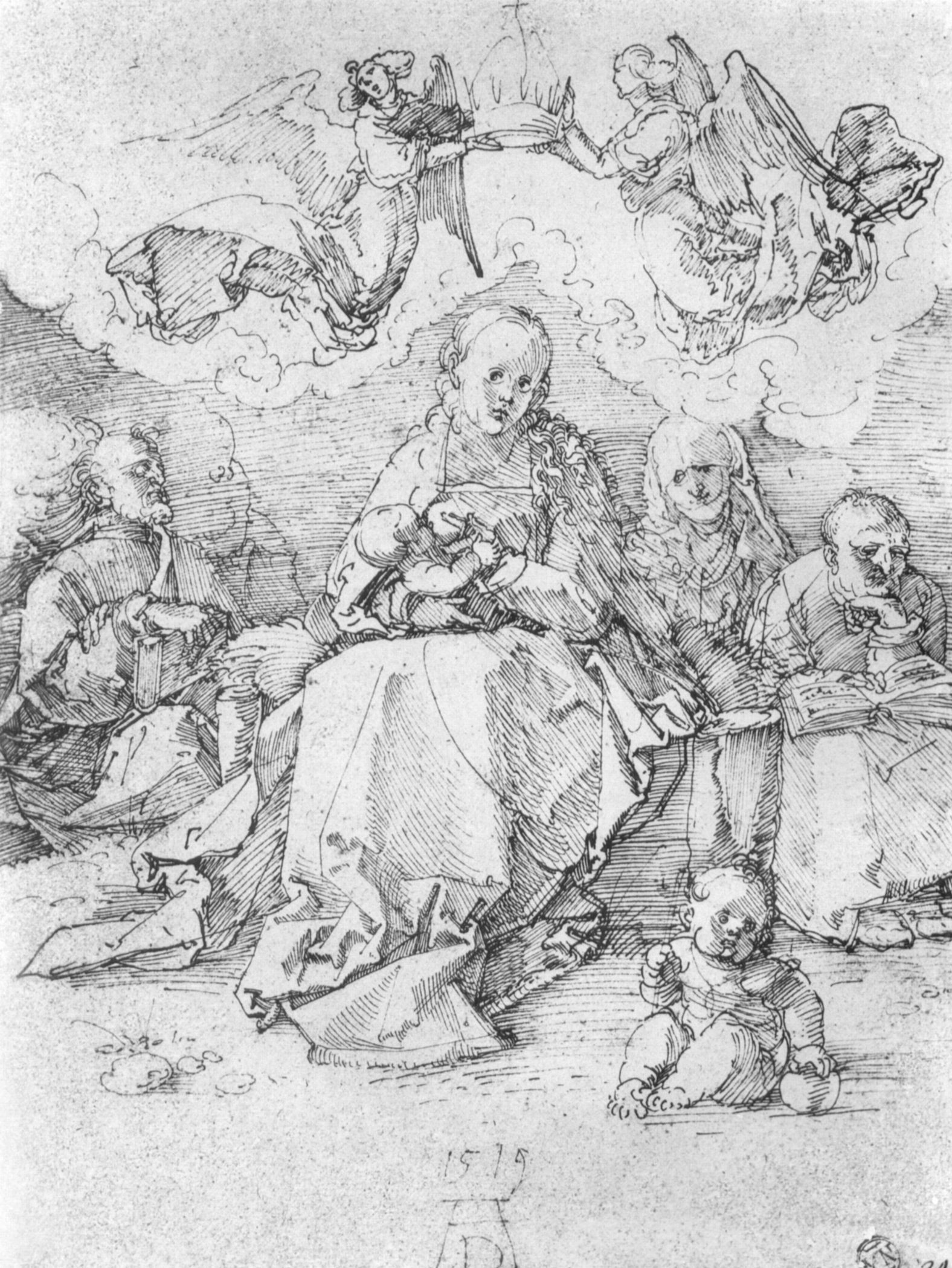This monochrome drawing, possibly a sketch or print from 1519, features a solemn indoor scene rendered in fine lines, suggesting it was created with pencil or graphite. At the center is a woman dressed in detailed robes, her expression weary as she tenderly suckles a newborn. To her left stands a robed man holding an open book, his gaze directed upwards in contemplation. Adjacent to him is an infant, barefoot and clutching a ball, who looks outward with a curious expression.

On the woman's right sits an older woman adorned in a headdress and robe, her face reflective. Further right, a bald older man kneels in front of an open book, his eyes lifted towards the central woman. Above them, two ethereal angels hover within the clouds, each gracefully extending a hand to hold a crown above the mother's head. The composition, potentially a religious depiction involving Mary and the baby Jesus, captures the varying emotions and intricate details of the figures' attire and surroundings with masterful precision.